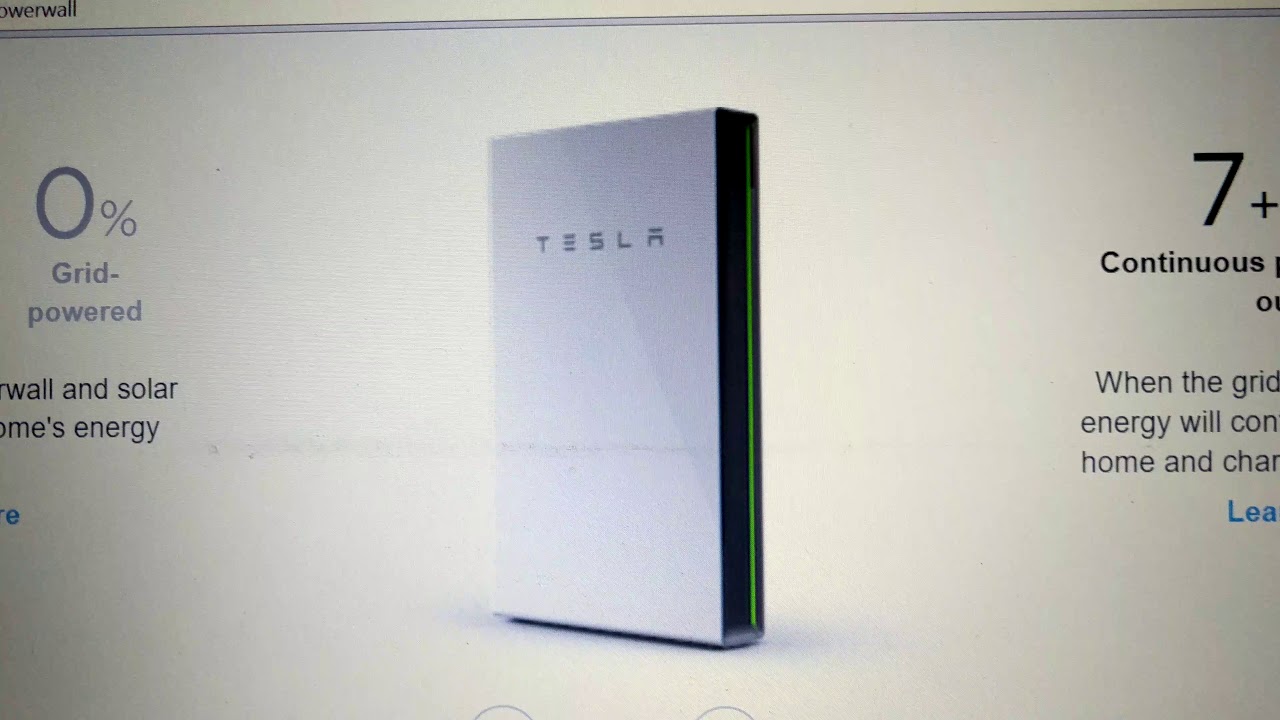The image displays a computer monitor with an open web page. In the top left corner of the screen, the words "Powerwall" are written as a single word in black font. Below this header, the web page has a lavender hue. Central to the image is a depiction of a Tesla Powerwall unit, characterized by a pastel purplish shade. A green line appears to the right of the unit, and there is a black section on the right side.

The visible text on the left side of the screen includes "0% grid powered." Additionally, it mentions "Powerwall and solar energy," though the text is partially cut off. On the right, the text begins with "7+" but is similarly incomplete. The fragmented text continues with phrases such as "when the grid," "energy will," "home and car," and "learn," although some portions are obscured or cut off.

Below this section, two partially visible buttons are situated—grey with a pastel lavender tone. They are cut off at the top, making full text unreadable. The overall layout prominently features the Tesla Powerwall product in the center of the screen, with the "Powerwall" label in the top left corner.